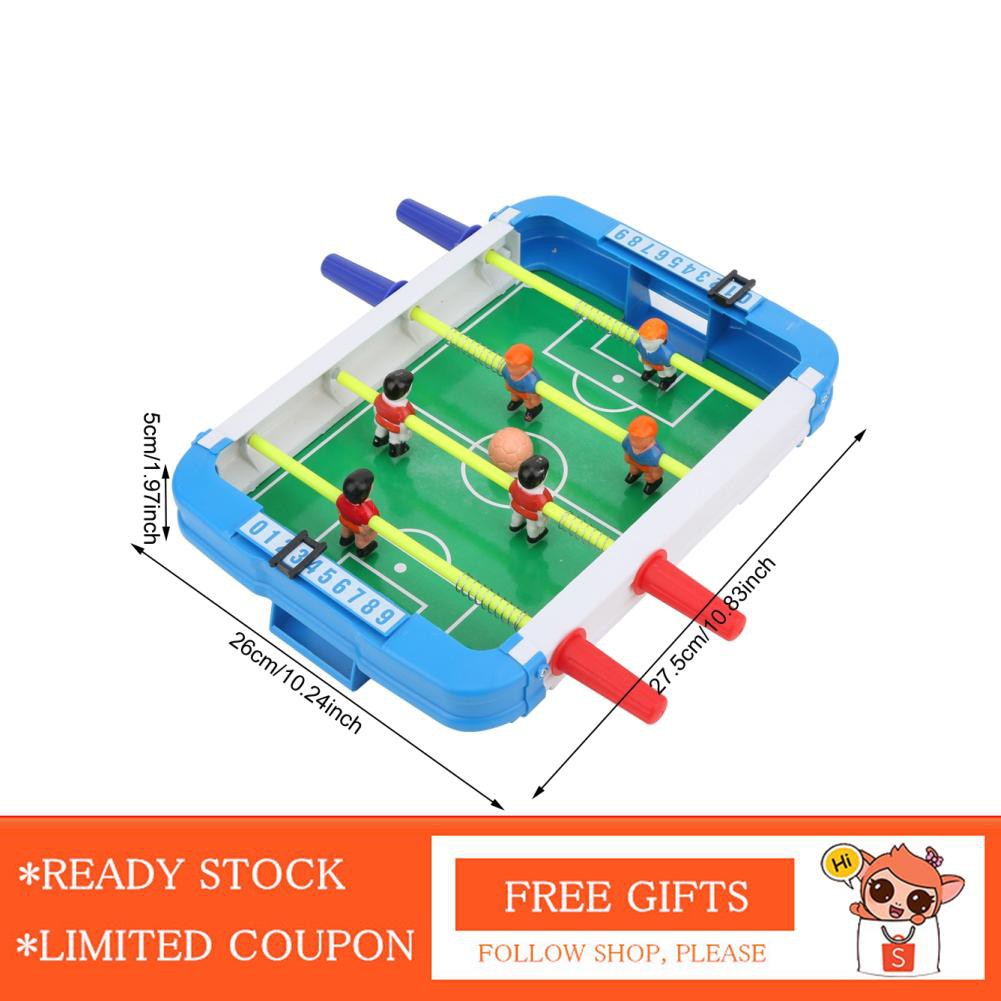In the image, a miniature foosball table takes center stage, tilted slightly to the right. The table features a green and blue field, surrounded by players in red, white, blue, and orange uniforms. The handles are on either side—green and blue on the right, and unspecified on the left—with yellow poles connecting them. At the bottom right, a small stuffed animal peeks out from a bag. The image includes an orange and white banner at the bottom, with text promoting "Ready Stock," "Limited Coupon," "Free Gifts," and "Follow Shop, Please" in white font. The overall setting appears to be an advertisement highlighting the dimensions, colors, and design of the foosball table.